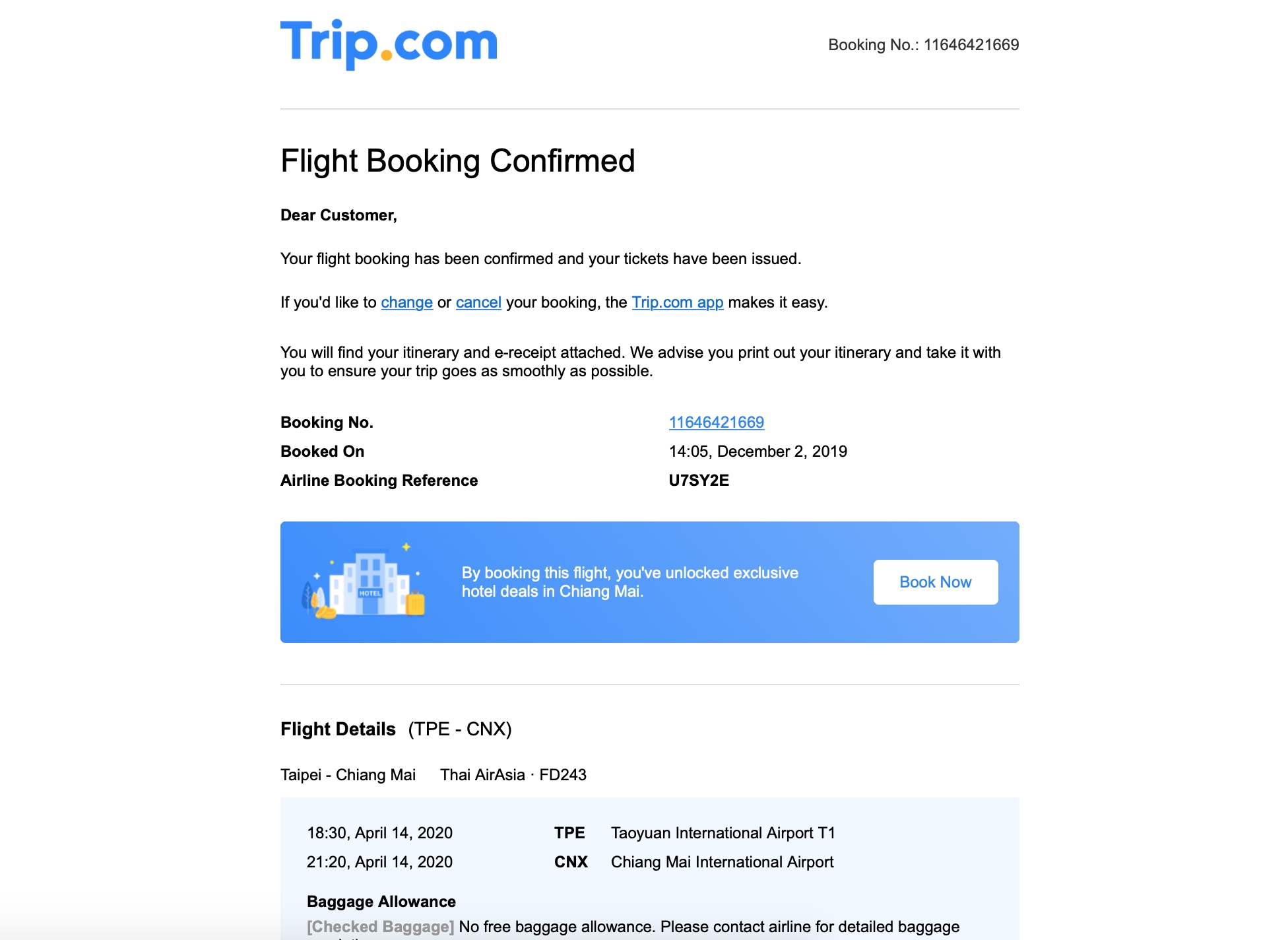The screenshot captures a website interface for Trip.com. At the top left corner, 'Trip.com' is displayed in distinctive colors: 'Trip' in blue, the dot in yellow, and the comma in blue. On the right side of this header, the Booking Number, 116-464-21669, is prominently shown against a white background, separated by a gray line below.

Just beneath this gray line, a bold headline reads "Flight Booking Confirmed." In smaller text underneath, a message to the customer states: "Dear Customer, your flight booking has been confirmed, and your tickets have been issued."

The next line introduces instructions for changes or cancellations: "If you'd like to change or cancel your booking, the Trip.com app makes it easy." This is followed by clickable, underlined links labeled "Change" and "Cancel on Trip.com" in blue.

Further down, an advisory section informs the customer: "You will find your itinerary and email receipt attached. We advise you to print out your itinerary and take it with you to ensure your trip goes as smoothly as possible."

Details of the booking are reiterated below this information, displaying the Booking Number 116-464-21669 once more, alongside the booking date and time, "Booked On: 1405, December 2nd, 2019," and the Airline Booking Reference: U7SY2E.

At the bottom of the page, a vivid blue bar highlights an enticing offer: "By booking this flight, you've unlocked exclusive hotel deals in Chiang Mai." This section is followed by a summary of the flight details.